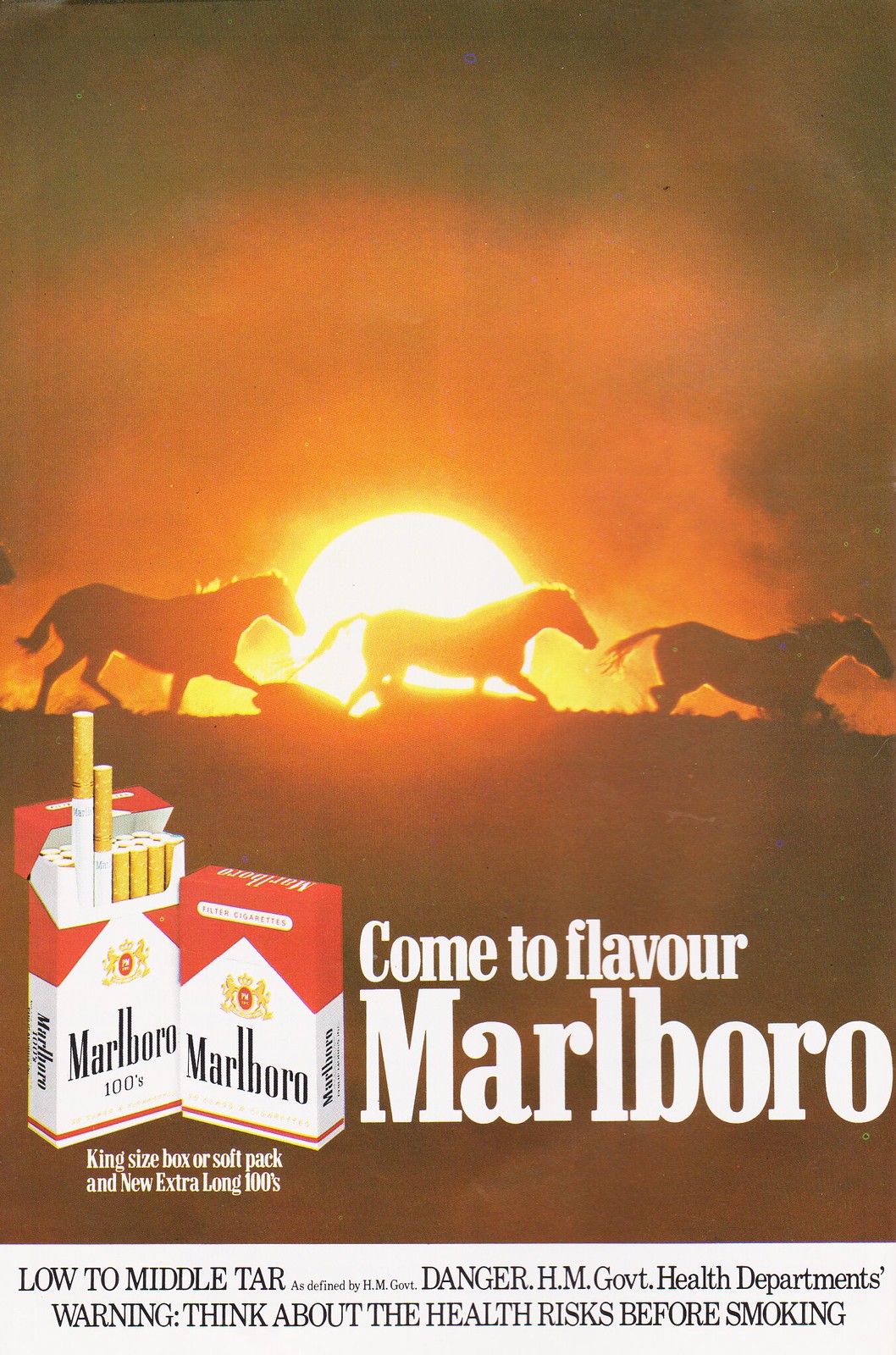This Marlboro cigarette advertisement is a visually striking poster set against a breathtaking sunset. Dominating the background is a radiant sun casting a golden glow across the horizon, transitioning the sky from bright yellow near the sun to a blend of deep burnt orange and reddish hues. Silhouetted against this vivid backdrop, three majestic horses gallop in a line, their manes and tails seemingly aflame with the sun's light as they move uphill across the open plain. 

In the lower left corner, there are two distinctive packs of Marlboro cigarettes, one open with cigarettes visible and the other closed. Both packs feature the iconic red top and white body, emblazoned with the black Marlboro logo. To the right of the packs, bold white text reads, "Come to Flavor Marlboro." Beneath this, additional text notes the options available: "King Size Box or Soft Pack and New Extra Long 100s." 

Framing the bottom of the advertisement, a gray border carries critical health information in black text: "Low to Middle Tar, as defined by HM Government, Danger, HM Government Health Department's Warning, Think About Health Risks Before Smoking." 

This carefully crafted composition effortlessly blends the allure of a serene natural setting with the branding and product information for Marlboro Cigarettes, all while ensuring the necessary health advisories are prominently displayed.